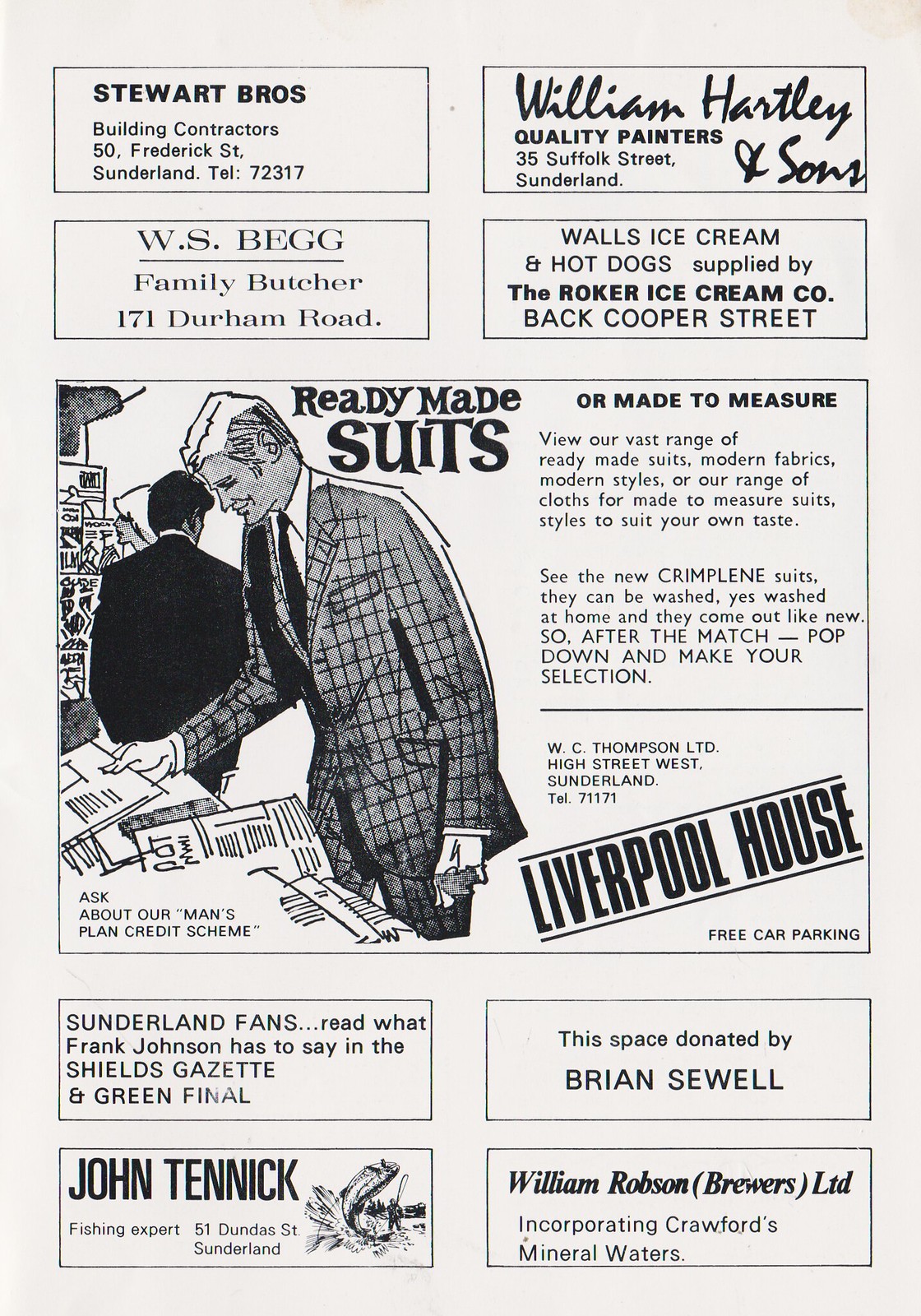This is a detailed black-and-white scan of an old advertisement page from a magazine or newspaper. The page is divided into multiple sections, showcasing various businesses. The top part has four quadrant boxes featuring ads for Stewart Brothers, building contractors; William Hartley & Sons, quality painters; W.S. Big, Family Butcher; and Walls Ice Cream and Hot Dogs supplied by the Roker Ice Cream Company.

At the center of the page, there's a large square illustration of a man dressed in a stylish suit with pinstripes and a tie, looking down at some papers or magazines. To his left, another man in a dark suit, seen from the back, is positioned in what appears to be a store with items on the shelf beside him. The illustration is accompanied by a promotional text for ready-made and made-to-measure suits, highlighting modern fabrics and styles, including the new Crimp line suits that can be washed at home and look like new. The text urges readers to visit after the match to explore their selection.

Below this central illustration, there are four more rectangular ads. One features an endorsement for Sunderland Fans by Frank Johnson in the Sheffield Grisette. Another ad states, "This space donated by Brian Sewell." Additionally, there's an ad for John Tennick, a fishing expert, and William Robeson Brewers Ltd., promoting their incorporation of Crawford's mineral waters.